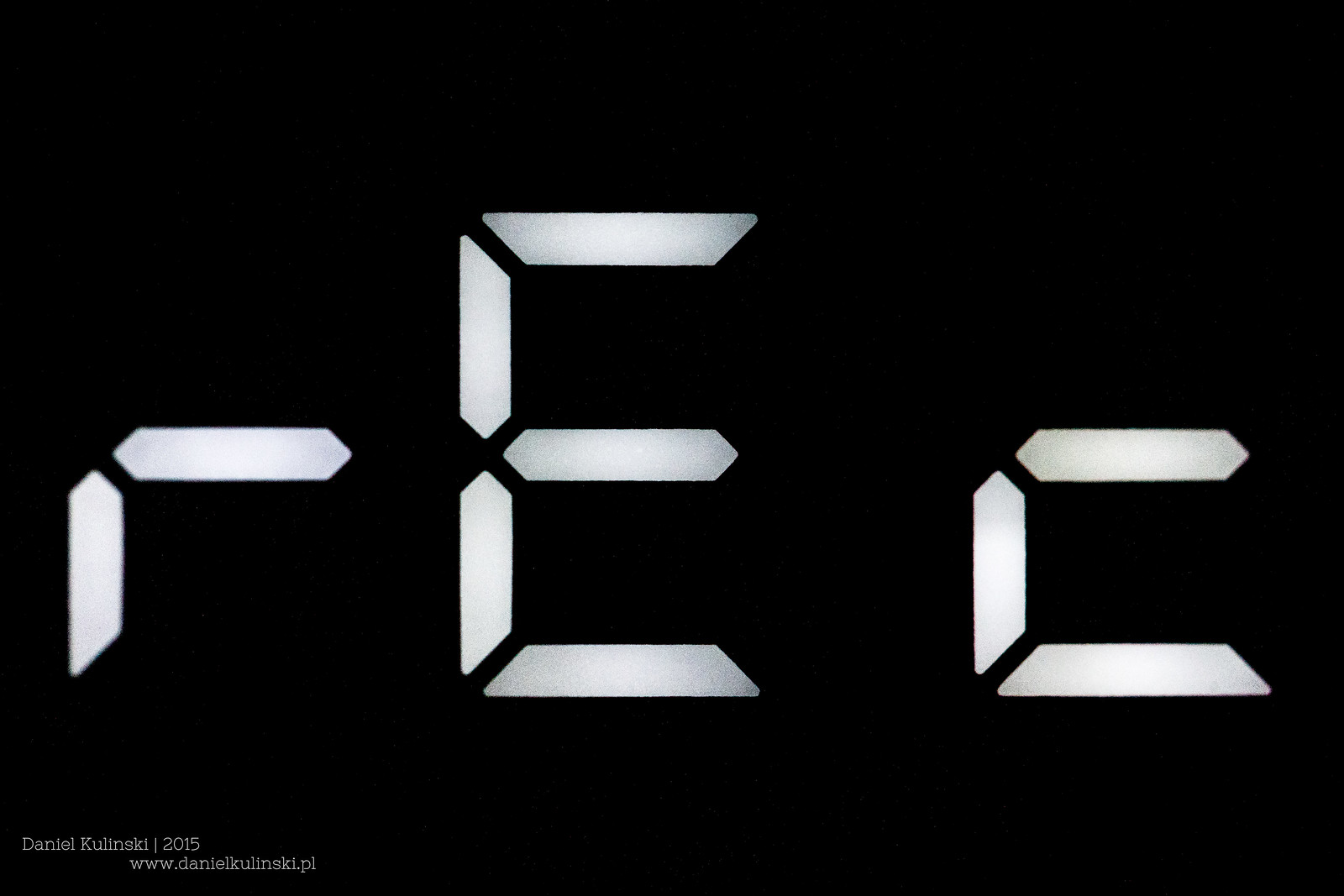In this black and white minimalist image, the background is rendered in deep black, providing a stark contrast to the elements in the forefront. In the lower left-hand corner, inscribed in small white print, is a credit line that reads "Carmel or Council Connock, 2015." Adjacent to this, part of a website address is visible, starting with "www." and ending with ".pl," suggesting it is likely a Polish website.

Centrally positioned are three abstract, digital-like symbols. The middle symbol is a white, incomplete digit reminiscent of the number '8' but appears more like a distorted 'E' due to the absence of the right-hand lines. To the left of this central symbol is an 'R'-like figure, characterized by a combination of short vertical and horizontal lines, the latter being aligned with the middle bar of the 'E'. On the right-hand side, a figure resembling a small 'C' mirrors the positioning with its horizontal line matching the middle bar of the 'E' as well. These symbols together create an intriguing, cryptic display, blending geometric simplicity with digital aesthetics.